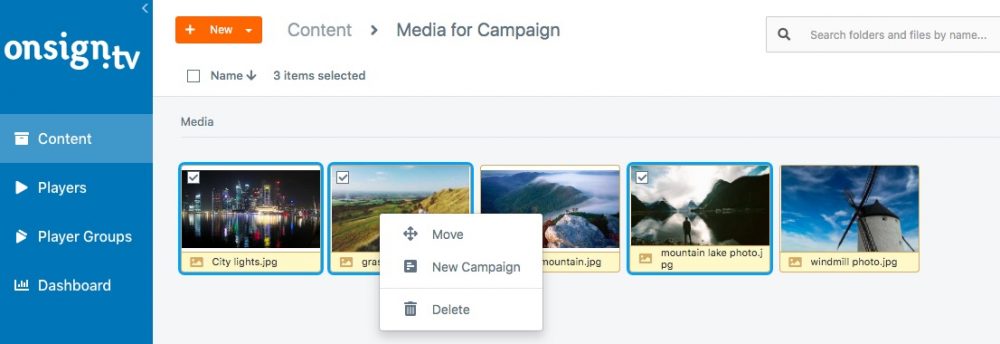The image displays the interface of the unsigned.tv application. On the left, a vertical menu set against a blue background features options in white text: "Content," "Players," "Player Group," and "Dashboard." The top of this menu prominently displays the application's name, "unsigned.tv." 

To the right, the interface is divided into sections. At the top, there is a row of actions labeled "New," followed by "Content," "Media," and "Campaign." Below this, a section titled "Name" indicates that three items are selected. A search bar located in the top right has the placeholder text "Search folders and files by name" and is set against a light grey background. The rest of the right side has a light white and grey color scheme.

In the media section at the bottom, five pictures are displayed, with three highlighted. The first image is titled "City Lights," showing city lights reflecting on a lake. The second image, labeled "Grass," depicts a green and yellow field of grass and is highlighted. The third image, "Mountains," features mist-covered mountains but is not highlighted. The fourth image, which is highlighted, shows a person facing a range of dark mountains under a cloudy sky, and is titled "Mountain." The final image, "Windmill Photo," shows a windmill set against a blue sky and white concrete surface.

Options to "Move," "New Campaign," or "Delete" appear at the bottom, corresponding to the highlighted items.